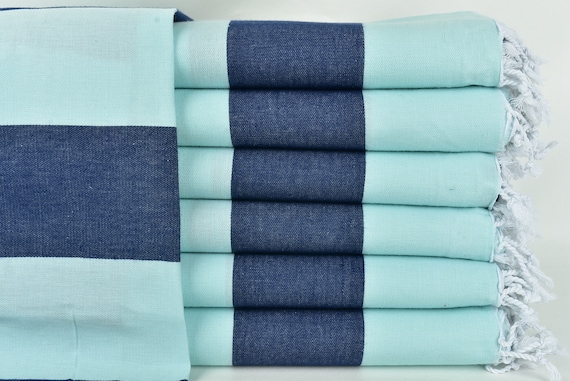This photograph depicts a neatly stacked pile of six aqua-colored textiles, which appear to be either beach towels or fringed blankets made of a natural material, possibly cotton. Each textile features a broad, dark denim blue stripe running down the center, flanked by a lighter aqua hue. A row of whitish aqua fringe lines the edges, adding a soft, decorative touch. One of the textiles on the left side is unfolded slightly, revealing more of its interior and the continuity of the dark blue stripe against the aqua background. The stack of textiles is set against a simple, light grayish-white backdrop, highlighting the even alignment of the stripes and the careful, organized presentation of the folded pieces.